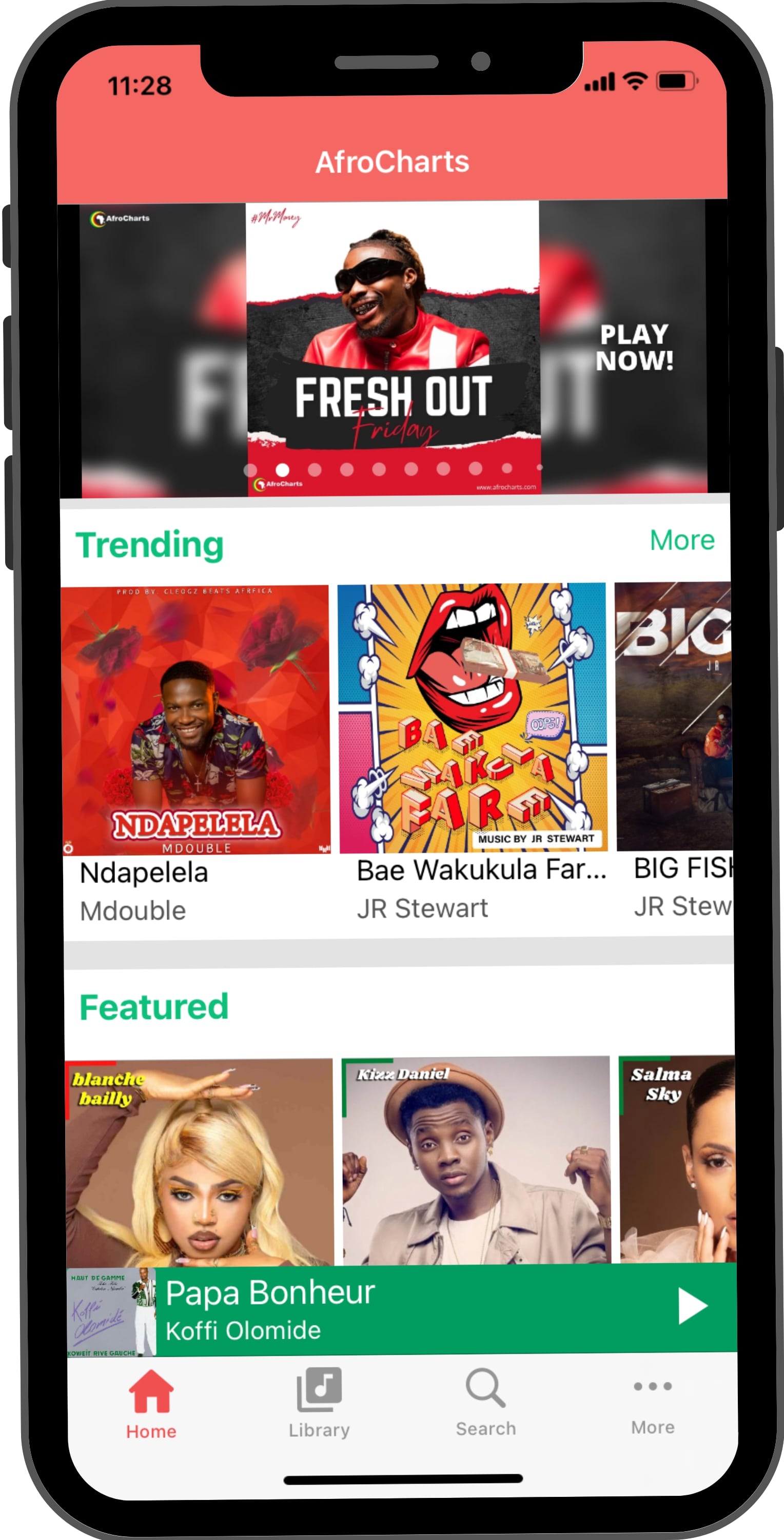The image depicts a black cell phone with a website display photoshopped onto its screen. The phone features three buttons on the left side and one on the right side. At the top, there's a grey bar in the center and a grey dot to the right. On the screen, the top left corner shows the time "11:28," and the top right corner displays a nearly full battery icon, WiFi connection, and full cell signal bars.

The top banner on the screen reads "Afrocharts" in white font against a salmon-colored background. Below the banner, there's an album section titled "Fresh Out Friday," displaying an album cover featuring a man in a red and white leather jacket and black sunglasses, smiling. The text "Play Now" appears in white font on the right side of this section. 

Further down, there are two sections: "Trending" and "Featured," each showcasing three album covers, with the option to scroll to view more. 

At the bottom of the screen, a green banner indicates the currently playing track, "Papa Bonheur Coffee Oloh Myed," alongside a play button and an album cover depicting a man wearing white pants and a button-up shirt, set against a purple background.